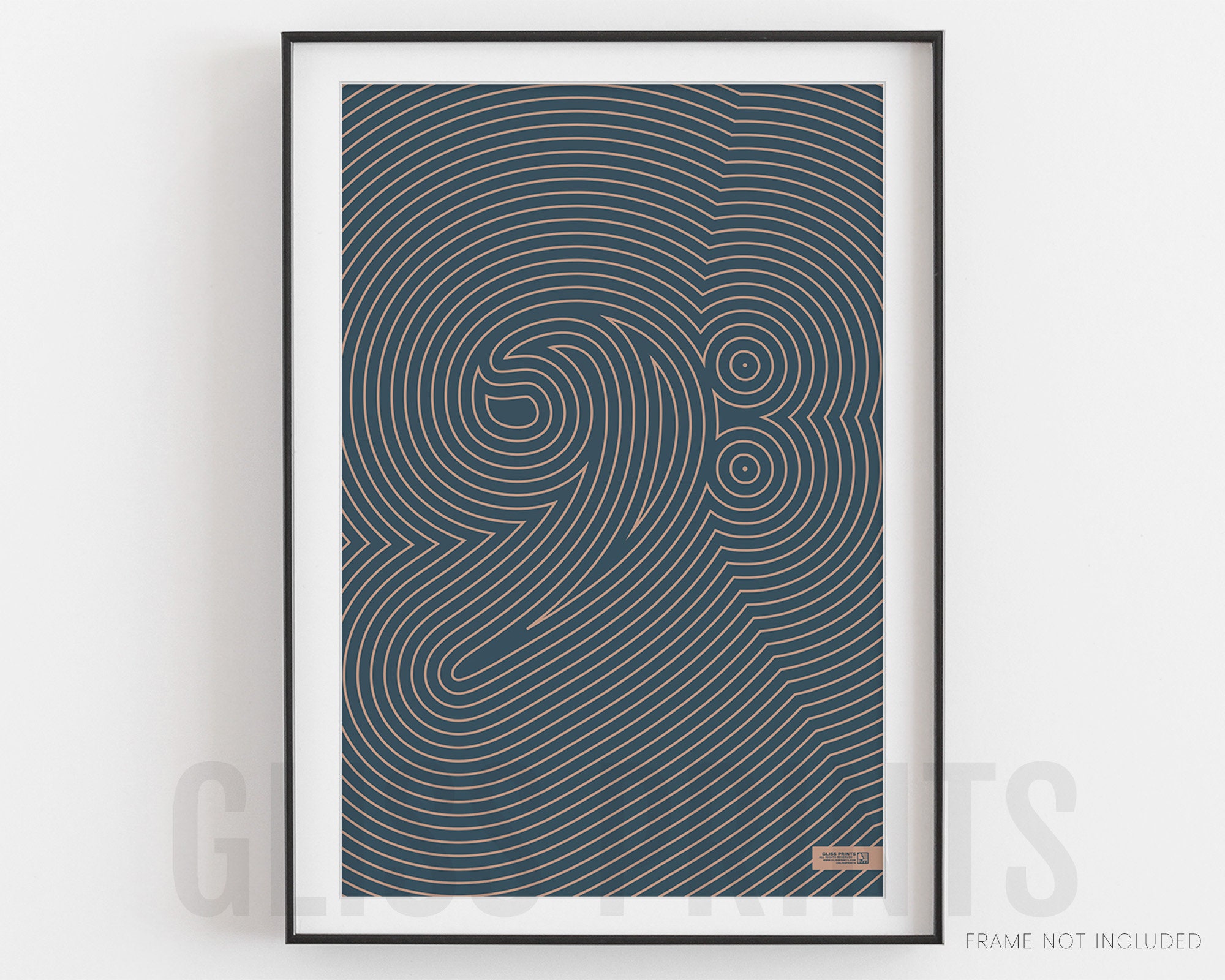The image depicts a framed piece of artwork set against a plain white background, creating a minimalist presentation suggestive of an online listing. The frame is slender and black, with a narrow white matting that borders the artwork. The picture showcases a geometric design on a dark blue background, characterized by intricate, non-intersecting beige lines that form concentric and circular patterns. Prominently, two circular shapes with distinct central points are positioned one above the other on the right side of the design. Transparent text across the bottom of the artwork reads "glass print," indicating a watermark to prevent unauthorized reproduction. Additionally, in the bottom right corner of the image, small all-caps lettering states "frame not included," clarifying that the frame is for display purposes only. The overall layout of the image, with the framed artwork centered against a white backdrop, emphasizes the aesthetic and commercial appeal of the piece.